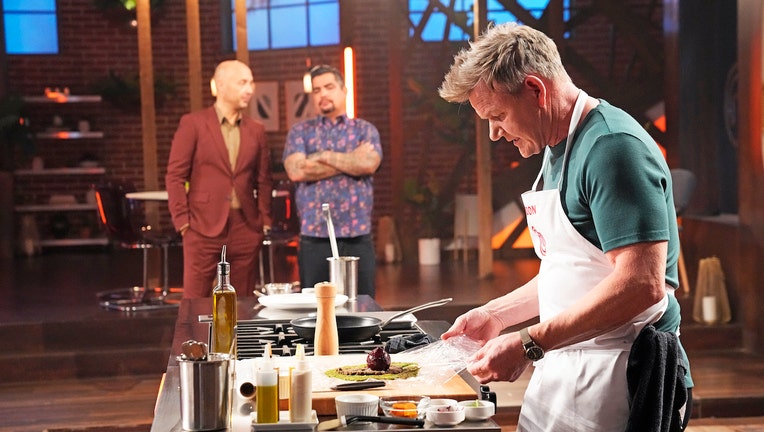In this detailed freeze-frame from the cooking show MasterChef USA, Chef Gordon Ramsay is prominently featured on the right side of the image, wearing a white MasterChef apron over a green short-sleeve shirt. He is looking down at a cooktop, preparing food with an assortment of cooking items in front of him. On the counter in front of Ramsay are scattered ingredients, including a bottle of olive oil, a salt and pepper shaker, small white and clear dishes with various spices, and a stainless steel canister holding utensils. A frying pan rests on the stove, and Ramsay appears to be handling cellophane, possibly to wrap the food he is preparing.

In the background, two other judges stand at the end of the cooking bench. Aaron Sanchez, dressed in a flowered shirt with dark pants and displaying tattoos on his forearms, stands with his arms crossed, observing Ramsay. Joe Bastianich, beside him, dons a rust-colored suit over a tan shirt and seems to be engaged in conversation with Sanchez. The set backdrop includes a brick wall, shelving, windows, and stairs, further grounding the scene in the familiar atmosphere of the MasterChef kitchen.